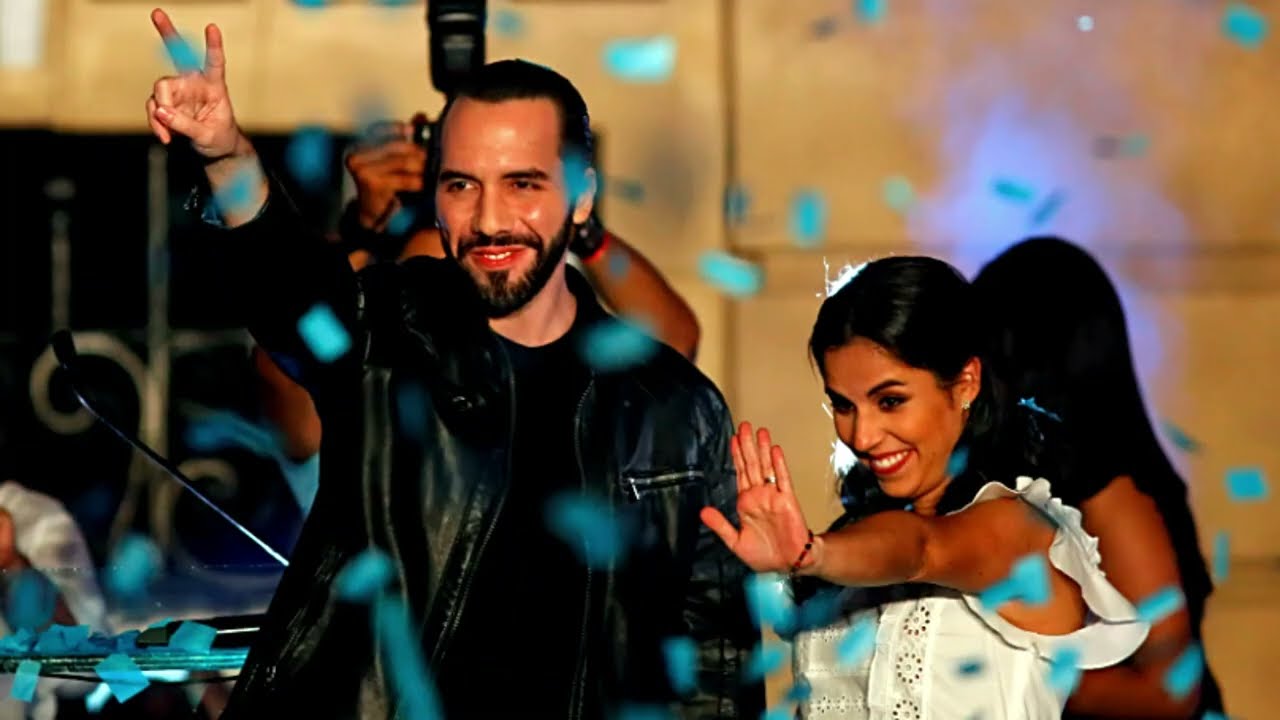In the image, two people are at the center, partially submerged in falling Tiffany blue-colored confetti. The man on the left wears a black leather jacket and a matching T-shirt. He has slicked-back black hair and a beard and mustache of the same color. He appears to be smiling and signaling a peace sign with his left hand. Beside him, on the right, stands a woman with long black hair and dark eyebrows. She has rich caramel-colored skin, red lips, and wears a white dress adorned with floral patterns. She appears to be waving with her left hand, displaying a gold ring on her fourth finger. Both individuals are positioned waist-up against a tan and black wall. Additionally, visible behind the man is a DJ booth with a microphone and turntable, suggesting a celebratory atmosphere, possibly a wedding.